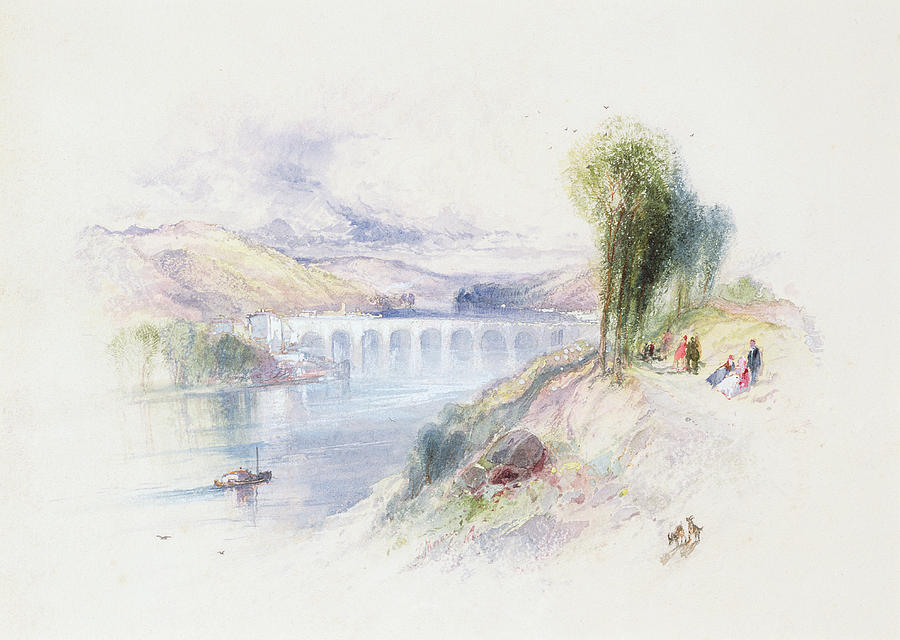This is a detailed watercolor painting with an off-white border, focusing the viewer's attention on the central scene. At the bottom right, a rocky hill-like surface transitions from light gray to a darker purplish gray, mingled with darker and lighter green areas peppered with small gray rocks. Atop this hill, several tall, bright green trees stand, their vibrant foliage contrasting sharply against the rocky terrain. Nearby, on light green grass, figures of people are scattered—some women in dresses and some men—enjoying the scene, with some of them lying down possibly on towels.

To the painting’s left, a serene body of water in light blue subtly reflects hues of white, blue, purple, and green, imbuing the scene with a tranquil, pastel quality. On the horizon, a long gray bridge, replete with several small tunnels, stretches across the scene, while a backdrop of rolling hills and a mountain range adds depth, their soft edges depicted in gentle tones of blue, purple, and light brown. Above, a scattering of puffy blue-tinged clouds completes the serene atmosphere.

Amidst this idyllic setting, two tiny dogs can be seen playing near the people, adding a touch of liveliness to the peaceful scene. The overall composition is bathed in a soft, pastel ambiance, with particular emphasis on the blend of light and vibrant colors, giving it a dreamy and serene quality.